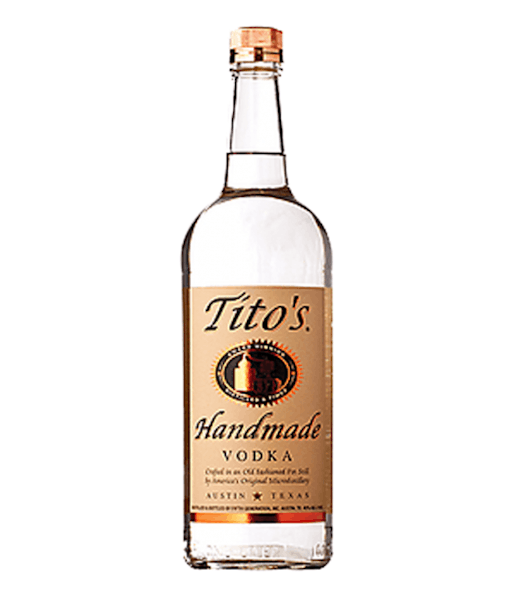The image features a clear bottle of Tito's Handmade Vodka standing upright against a white background. The bottle is topped with an orange, brass-like screw-on cap. The label, which occupies about three-quarters of the bottle, is predominantly an orange-brown color. "Tito's" is written in italic black letters at the top of the label, followed by a circular, black, oval-like logo underneath. Below the logo, "Handmade" is written in italic letters, while "Vodka" appears in plain font. The bottom of the label reads "Austin, Texas", flanked by a black star. The overall presentation is simple, with no shadows adding to the minimalist aesthetic.